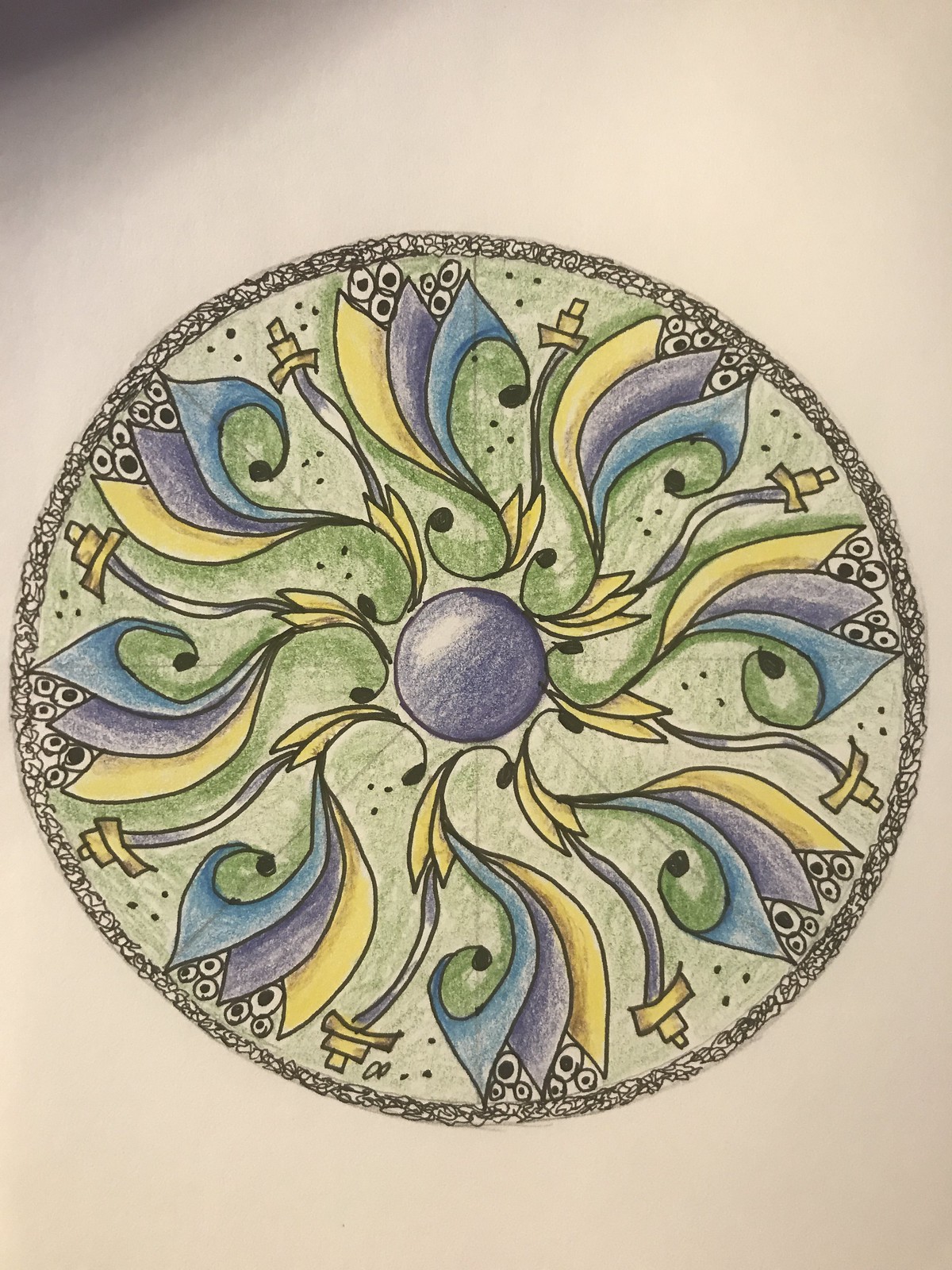This image features a meticulously detailed crayon drawing, presented against a gradient background blending shades of purple and white. The drawing itself is circular with a border composed of evenly spaced black dots. The main face of the circle is colored in light green, while the center contains a prominent purple circle. The design is characterized by its symmetrical patterning, including intricate motifs such as a repetitive yellow, purple, and blue swirl, and a sword-like shape pointing downwards. This sword design is repeated eight times around the circumference of the circle, adding to the overall symmetry and aesthetic harmony of the artwork.